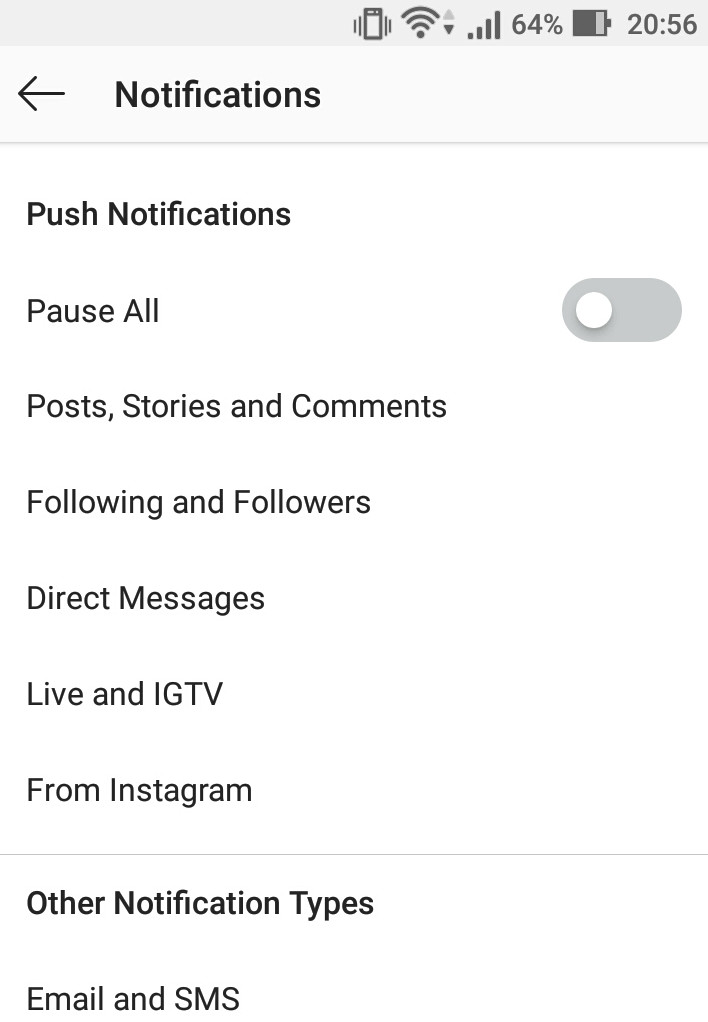This black-and-white screenshot, presumably taken from a phone, showcases the notifications area. At the top, a light gray banner is visible, housing various icons from left to right: a phone toggle, a Wi-Fi icon, a down arrow highlighted darkly against an up arrow, full signal bars, a 64% battery indicator, and the military time, 20:56. Below the banner on the left, an arrow points leftward next to the word "Notifications" in bold. Underneath, "Push Notifications" is prominently displayed in bold text, followed by the option to "Pause All," accompanied by a toggle button set to off on the right. The options below, listed from left to right, include "Post Stories and Comments," "Following and Followers," "Direct Messages," and "Live and IGTV," each separated by a thin line. The lower section reads "From Instagram," with another thin line separating the following text. Highlighted in bold once more, "Other Notification Types" is followed by "Email and SMS," completing the detailed enumeration of notification settings available in this capture.